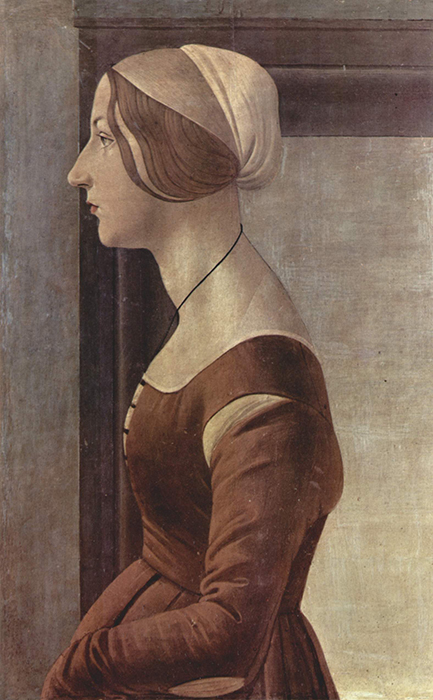The image depicts a detailed and vivid oil painting of a woman facing left, rendered with careful attention to profile and period styling. She has a long, pale neck and her nose appears pronounced, giving her an aristocratic air. Her lips, accentuated with red lipstick, contribute to her striking facial features. The woman has brown hair, partially covered by a beige headdress that transitions to white fabric at the back, with strands of her hair spilling out subtly. 

She is adorned with a thin, black string necklace that delicately wraps around her elongated neck. Her attire consists of a tight-fitting brown satin dress that hugs her torso, characterized by lines around the chest and shoulders, and then billows out towards the bottom, suggesting a period piece with a suede texture. Behind her, a dark brown wooden doorway frames her figure, contrasting with the gray wall to the left and transitioning to lighter brown and beige hues within the doorway space. The painting's clear and bright lighting, coupled with a noticeable light source from the lower right, illuminates the woman, giving a crisp, vivid quality to the overall image.